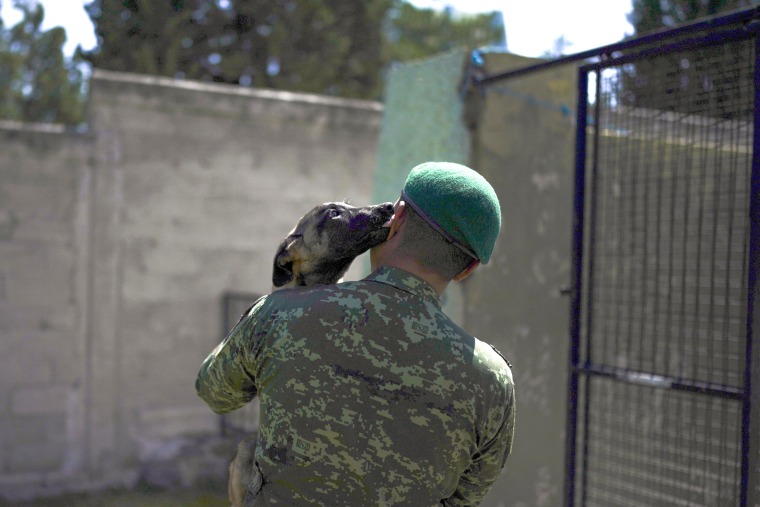In this image, we see the back of a muscular soldier dressed in digital camouflage uniform, predominantly featuring shades of green, brown, and black. He wears a distinguishing green beret, indicating he could be a member of a special forces unit. The soldier’s short-cropped hair is visible as he tilts slightly to the right, allowing a small brown and black dog, likely a Belgian Malinois, to affectionately lick his ear. The man cradles the dog in his arms, showing a moment of genuine joy and connection between them. Surrounding them is a fenced area with large greenish concrete walls and trees visible beyond the barrier, suggesting an outdoor setting during the daytime. To the right of the soldier, there is a black gate, possibly part of a dog kennel. The background appears slightly blurred, maintaining the focus on the touching interaction between the soldier and his loyal canine companion.